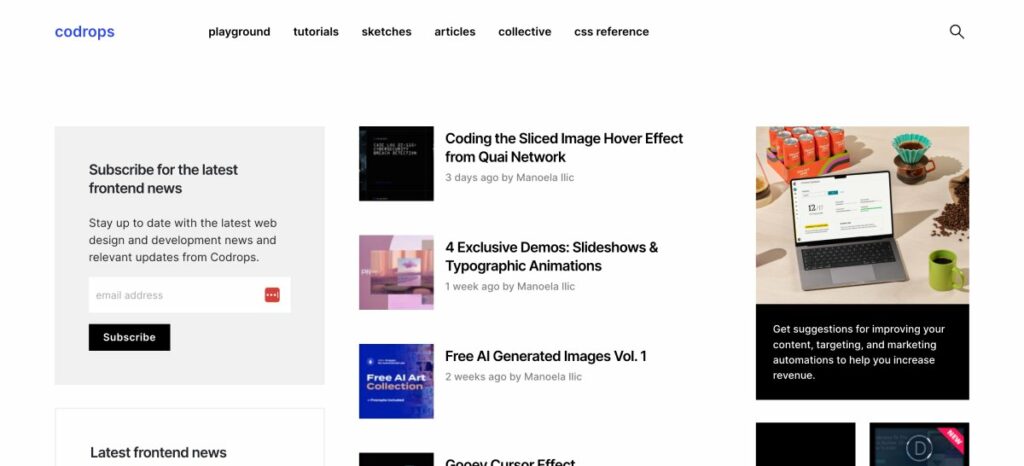The CO Drops homepage features a blue header with the site name at the top left corner. Directly beneath this, a black navigation bar runs across the screen, displaying tabs labeled Playgrounds, Tutorials, Sketches, Articles, Collective, and CSS Reference.

On the left side of the page, a gray sidebar invites users to subscribe for the latest front-end news. In this section, black text encourages visitors to "Stay up to date with the latest web design and development news and relevant updates from CO Drops." Below this call to action, a white input box labeled "Email Address" sits above a black "Subscribe" button.

Right under the subscription area, the sidebar's next section showcases the "Latest Front-End News." Adjacent to this, article links are prominently displayed. The first article, titled "Coding the Sliced Image Hover Effect from Quiet Network," was posted three days ago by Manoela Ilic. The article preview includes a black background with text indicating it covers exclusive demos, slideshows, and typographic animations.

A subsequent article, "Free AI Generated Images Volume One," is highlighted inside a blue box that reads "Free AI Art Collection." To the right of this, an accompanying image depicts a laptop alongside some drinks, suggesting content related to improving content targeting and marketing automations to help increase revenue.